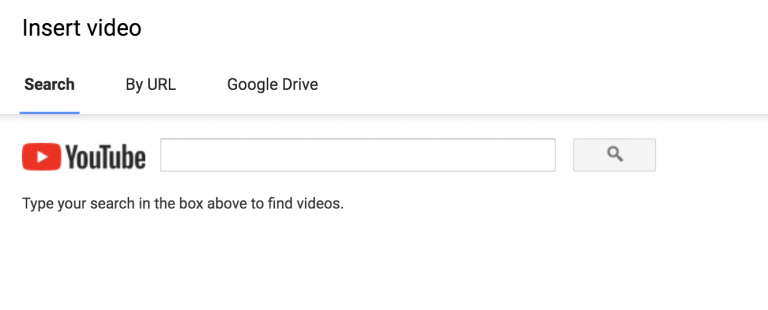This is a partial screenshot of a YouTube page. At the top, there is an inserted video surrounded by a black frame on a white background. Below the video, a menu strip is displayed, also with black text on a white background. The menu strip features several options, with "Search by URL" being the selected one and highlighted in bold. Next to it, another link labeled "Google Drive" is visible. The main section under the menu strip focuses on the search tab, which is currently active.

In this section, there is a central search box with the iconic YouTube logo positioned to the left of it. The search box itself is prominently placed in the middle, featuring a light gray rectangular search button with a small magnifying glass icon, signifying its purpose. Directly below the search box, there is an instructional message in plain text that reads, "Type your search in the box above to find videos."